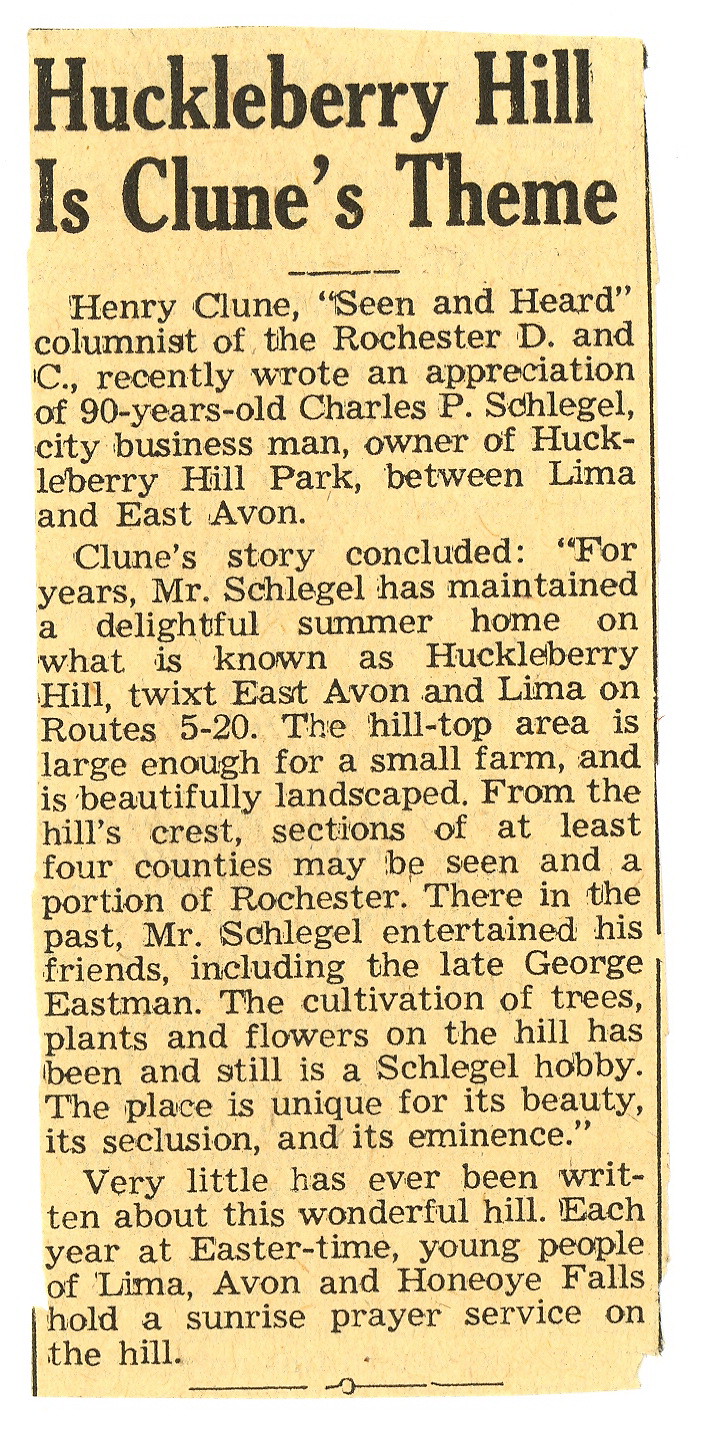The image is a yellowed newspaper clipping with the headline, "Huckleberry Hill is Clune's Theme." This article, written by Henry Clune, columnist of the Rochester D&C, celebrates Charles P. Schlegel, a 90-year-old city businessman who owns Huckleberry Hill Farm between Lima and East Avon. The piece details Schlegel's delightful summer home on Huckleberry Hill, situated on routes 5 and 20. The hilltop area, large enough for a small farm, offers a beautifully landscaped view from its crest. The article notes that very little has been written about this remarkable hill, where each year at Easter, young people from Lima, Avon, and Honeyoe Falls gather for a sunrise prayer service.